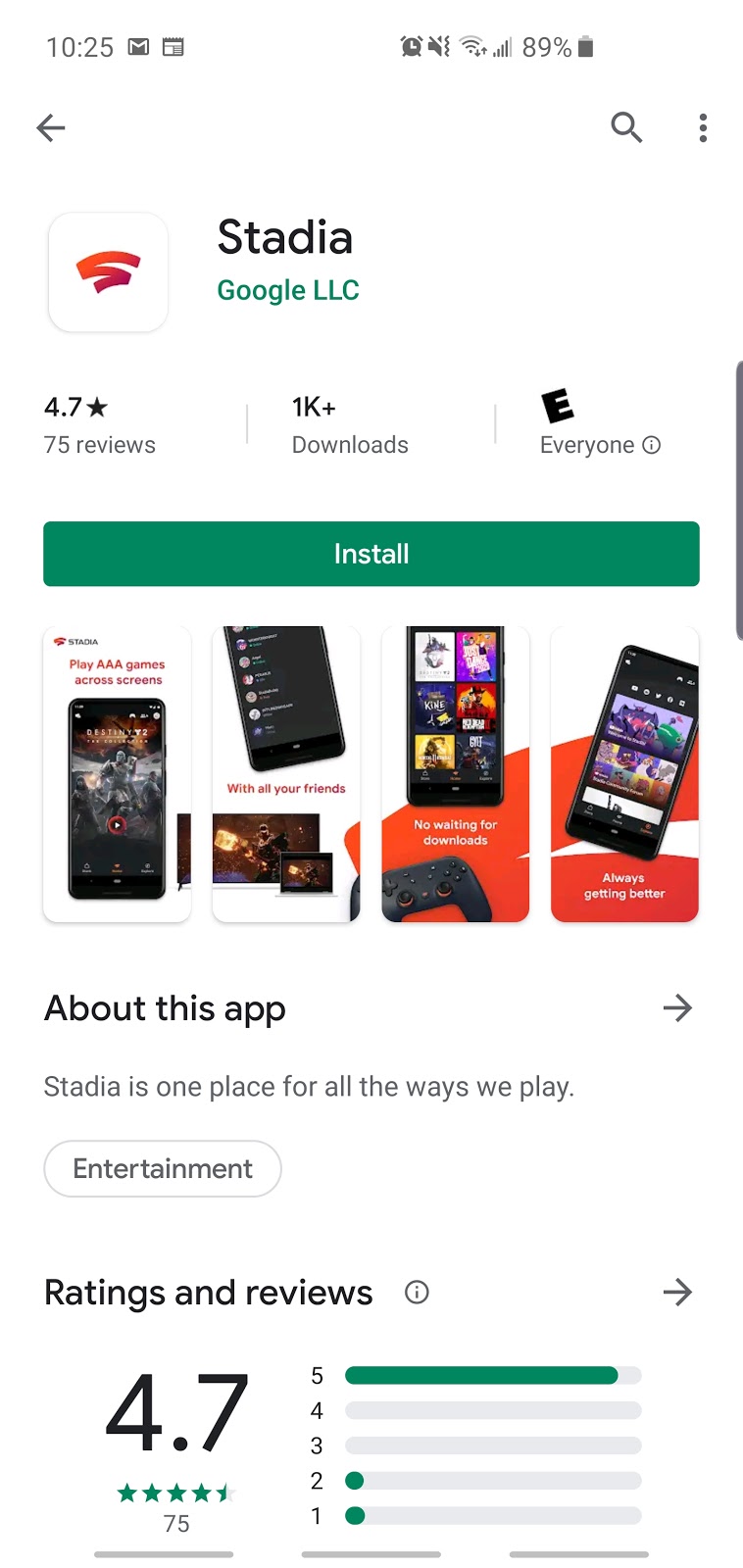In this image, the Google Play Store app interface for Android devices is displayed prominently. At the top of the screen, the status bar shows the time as 10:25 AM on the left, while the right side features icons indicating Wi-Fi signal strength, network signal, and battery level. The main focus of the interface is the Stadia app by Google LLC. The app boasts a 4.7-star rating, based on 75 reviews, and has achieved over 1,000 downloads. Additionally, it is rated appropriate for all ages.